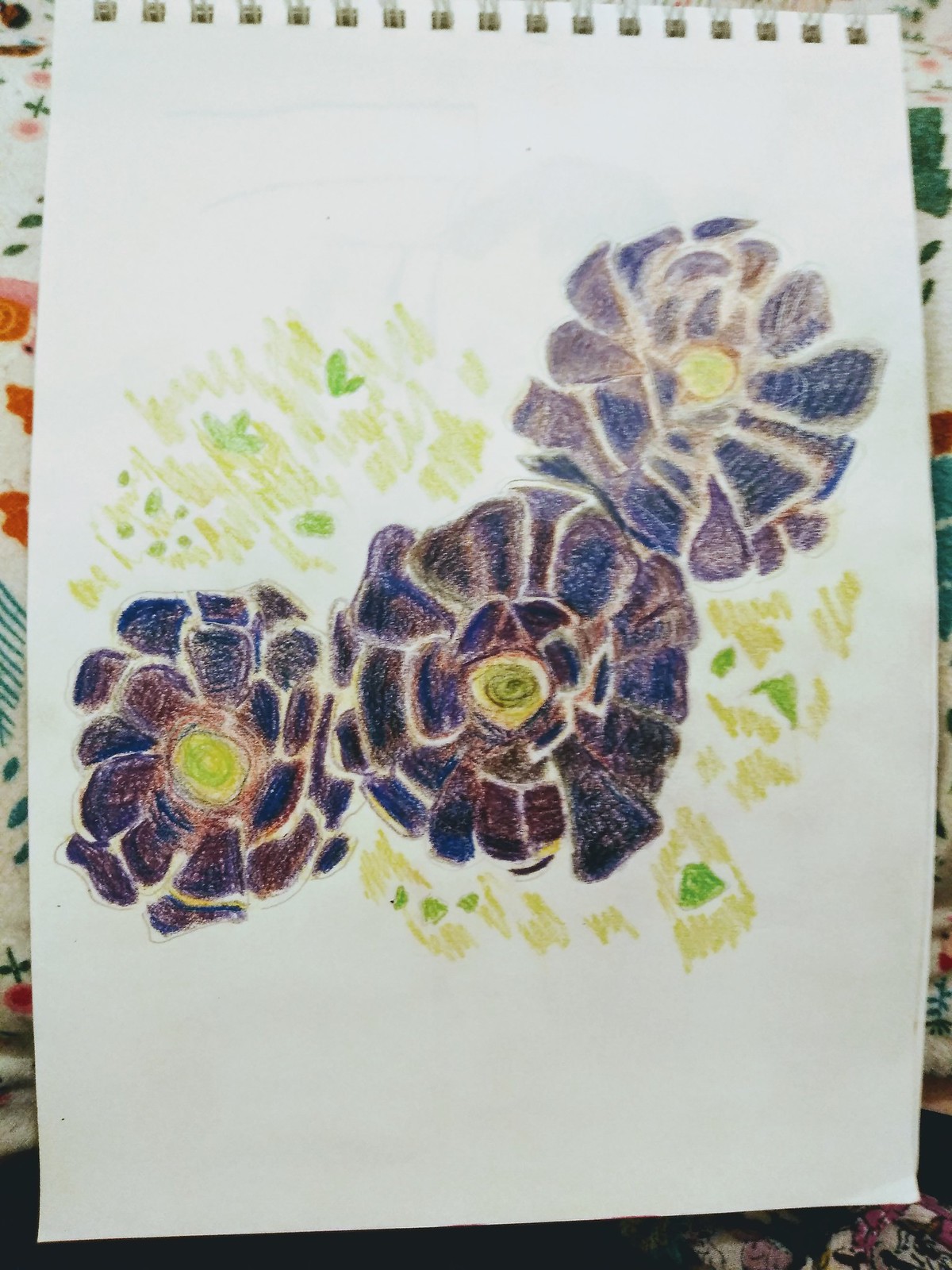A photograph captures a sketchbook set against a backdrop of a larger artwork or a mural. The sketchbook itself is the main focus, displaying a colored pencil drawing of purplish flowers with multitudes of petals and yellow centers. The backdrop adds depth to the composition, featuring a vibrant array of green and orange hues with pen markings and flowery patterns in the bottom right corner. The floral drawing in the sketchbook is complemented by grassy greens and yellow ochre shades in the background, showcasing a blend of purples, dark blues, and cranberry colors. The artwork has a charmingly simple and elementary style, reminiscent of a junior high classroom sketch.